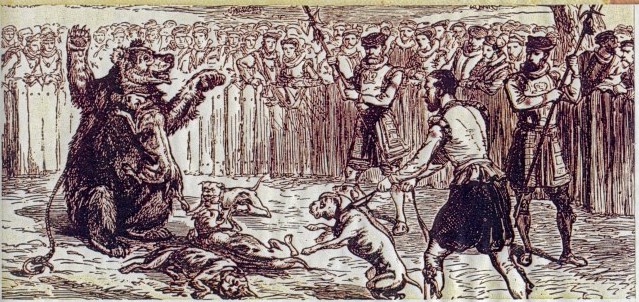The image is a detailed black and white, possibly brown and white, illustration resembling a scene from roughly 500 years ago. On the left side, a large bear, seemingly tied up, faces a few small dogs, with a couple lying down in the foreground. To the right, a person holds two dogs on leashes, attempting to restrain them, while two soldiers in armor, holding long spears, stand nearby. The scene appears chaotic, with the soldiers adding a hint of medieval or combat context. A wooden fence spans the horizontal middle of the image, separating hundreds of onlookers in the background, suggesting they are observing some form of public spectacle. The artistic medium, possibly pencil, pen, or charcoal, adds a classic, historical feel to the chaotic event.